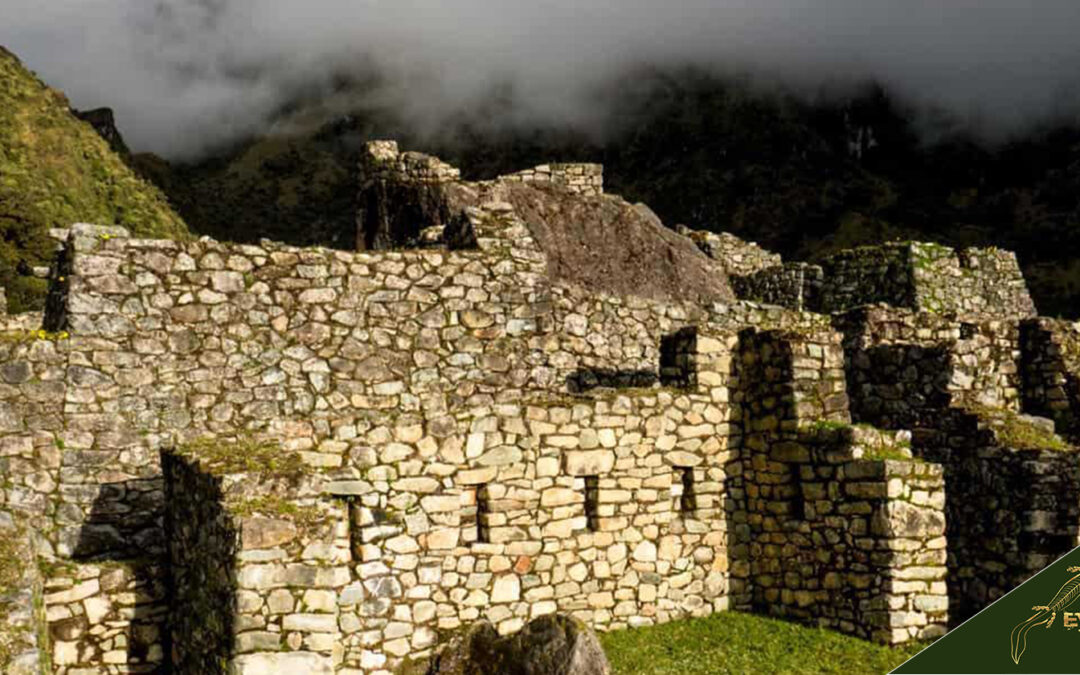This photograph captures an ancient, weathered stone structure set against a backdrop of mountains partially obscured by low-lying clouds. The structure, possibly the remnants of a castle or village walls, features intricately pressed stones of various sizes, assembled without mortar. The surfaces are marked by countless crevices where grass and low bushes have taken root, indicating a warm climate, perhaps in spring or fall. 

The main walls, which still stand upright, display an array of beige and light brown stones. The foreground wall, closer to the viewer, showcases a row of vertically aligned rectangular openings, likely windows, creating shadows within. Above and behind it, a taller wall with similar stonework looms, partially covered by a grayish, rectangular patch of what seems to be dry grass, masking the stone texture. 

To the left, the lower wall ascends initially at an almost right angle before sharply descending into steplike formations. Shadows cast in the corners of these angles hint at the light source originating from the upper left of the image. Pyramidal stone structures in the background appear truncated, adding to the ancient and enigmatic feel of the site.

The scene's periphery features a green expanse of rocky, grass-covered hills that blend into the mist-clad mountains, enhancing the mystical atmosphere. In the photograph’s bottom right corner, a cut-off green segment adorned with yellow designs resembles a finely drawn hand, potentially Tinker Bell’s, adding a curious, whimsical touch to the otherwise historical and archaeological ambiance.